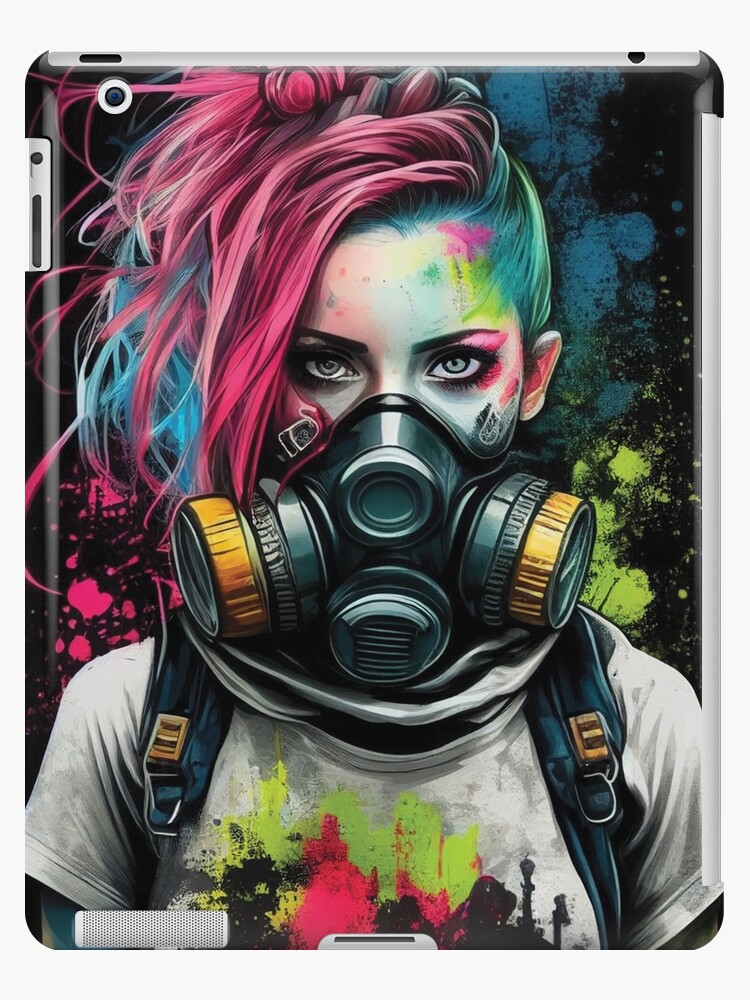This detailed tablet case features a vivid and colorful drawing of a post-apocalyptic scene. At its center is a woman staring directly at the viewer with piercing bluish-gray eyes. She wears a dark gas mask accented with orange, protecting her nose and mouth, suggesting she is in an environment with toxic air. Her long hair, styled to one side, is predominantly pink with streaks of blue and light green, and her face and hair are splattered as if she has been in a paintball fight or engaged in some form of street art. She wears a gray t-shirt adorned with abstract splotches of light green, pink, and black, which mirror the colorful splashes on her face and in her hair.

Adding to her rugged look, she dons a backpack with visible blue straps and possibly orange buckles. She stands against a black background that features random, vibrant splotches of blue, green, and pink, enhancing the chaotic, artistic vibe of the piece. The tablet case also shows details such as the camera and controls around the perimeter, seamlessly fitting the protector while showcasing this striking image.